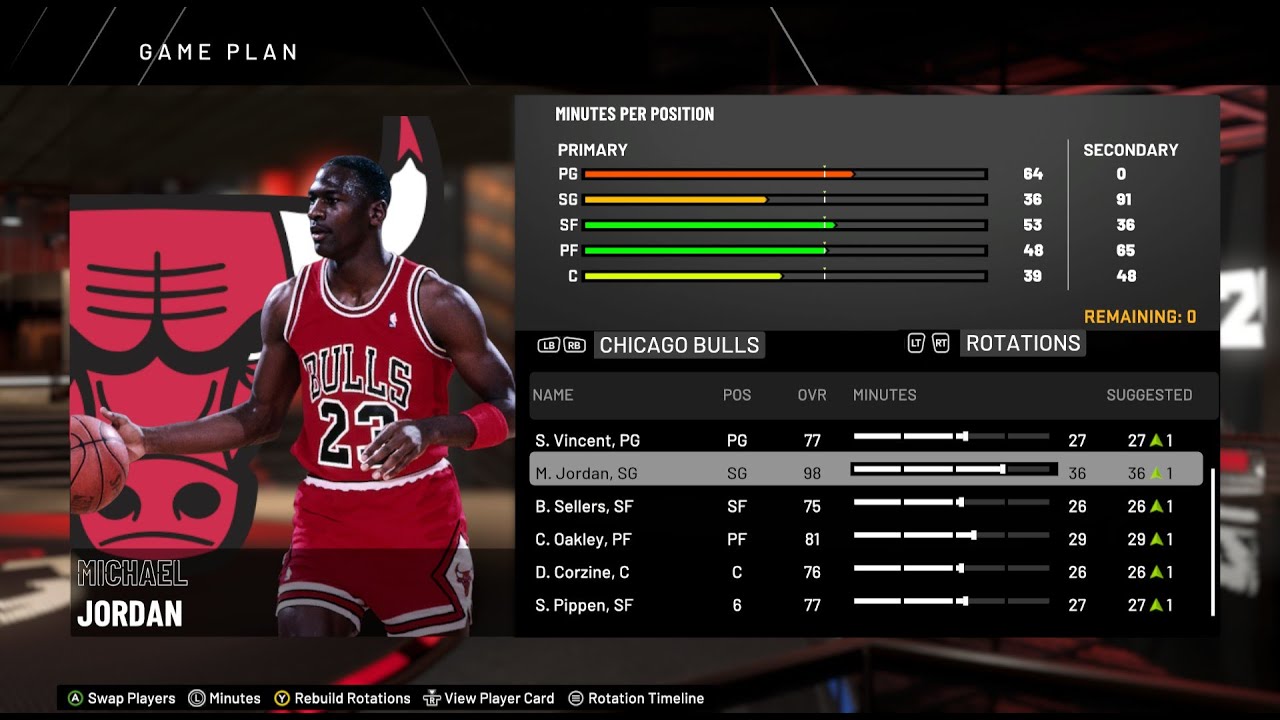Screenshot of a Basketball Video Game Interface – Chicago Bulls Game Plan

The image features a detailed interface from a basketball video game with a predominantly black background. Red, black, and white assorted logos populate the background, creating a visually engaging scene. Dominating the top-left corner of the screen, the word "GAMEPLAN" is prominently displayed in all caps with bold white text. Beneath this title, the iconic Chicago Bulls logo is prominently featured.

To the right of the logo, the legendary basketball player Michael Jordan is depicted wearing his signature Chicago Bulls #23 jersey in red and white. His name, "Michael Jordan," is displayed beneath his image to let players know who he is.

Adjacent to Michael Jordan's image, a gray box outlines the "MINUTES PER POSITION" in white text. This section provides a detailed breakdown of player positions and their allotted minutes. The positions listed include:
- PG (Point Guard) with an orange graph bar
- SG (Shooting Guard) with a yellow graph bar
- SF (Small Forward) with a green graph bar
- PF (Power Forward) with a green graph bar
- C (Center) with a yellow graph bar

To the right of these positions, respective numerical values for each position are provided: 64, 36, 53, 48, and 39. A vertical line separates this primary information from the secondary allocations which follow the same positional format with numerical values: 0, 91, 36, 65, and 48. The remaining value is noted as 0.

Below these data points, a black box provides additional navigational information, displaying "LBRB Chicago Bulls LTRT Rotations." Further detailed information is presented below, indicating elements such as "NAME PLS OVR MINUTES ADJUSTED" in support of player management and game strategy. A list of player names accompanied by a corresponding minute graph completes this comprehensive interface, allowing players to fine-tune team rotations and overall game plans.

This intricate screenshot encapsulates the strategic elements of managing the Chicago Bulls within the game, highlighting both visual and data-driven aspects crucial for gameplay.